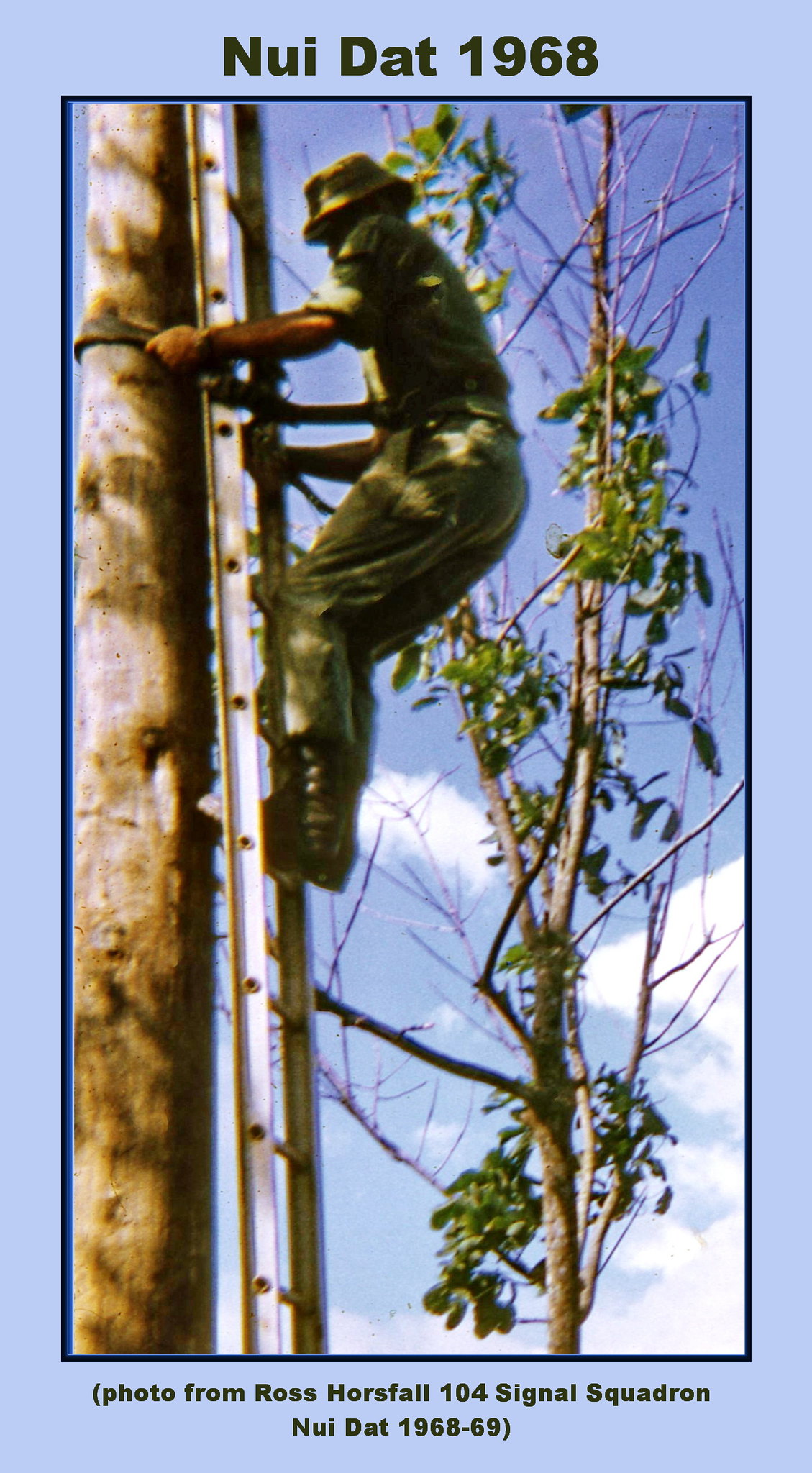This vertical, rectangular image from 1968 captures a man in a green army outfit—comprising olive green pants, shirt, bucket hat, and black boots—climbing a very tall tree or possibly a pole. He's using a long, silver ladder against the tree and is secured by a black leather strap around the trunk. The photo is framed by a light blue, sky-colored border, and you can see a thin tree with green leaves to the right. At the top of the image in dark green or dark gray font is the caption "Nui Dat 1968," and at the bottom, also in dark green font, it reads "photo from Ross Norsefall, 104 Signal Squadron, Nui Dat 1968-69." The background is a clear blue sky, indicating the height at which the man is positioned.